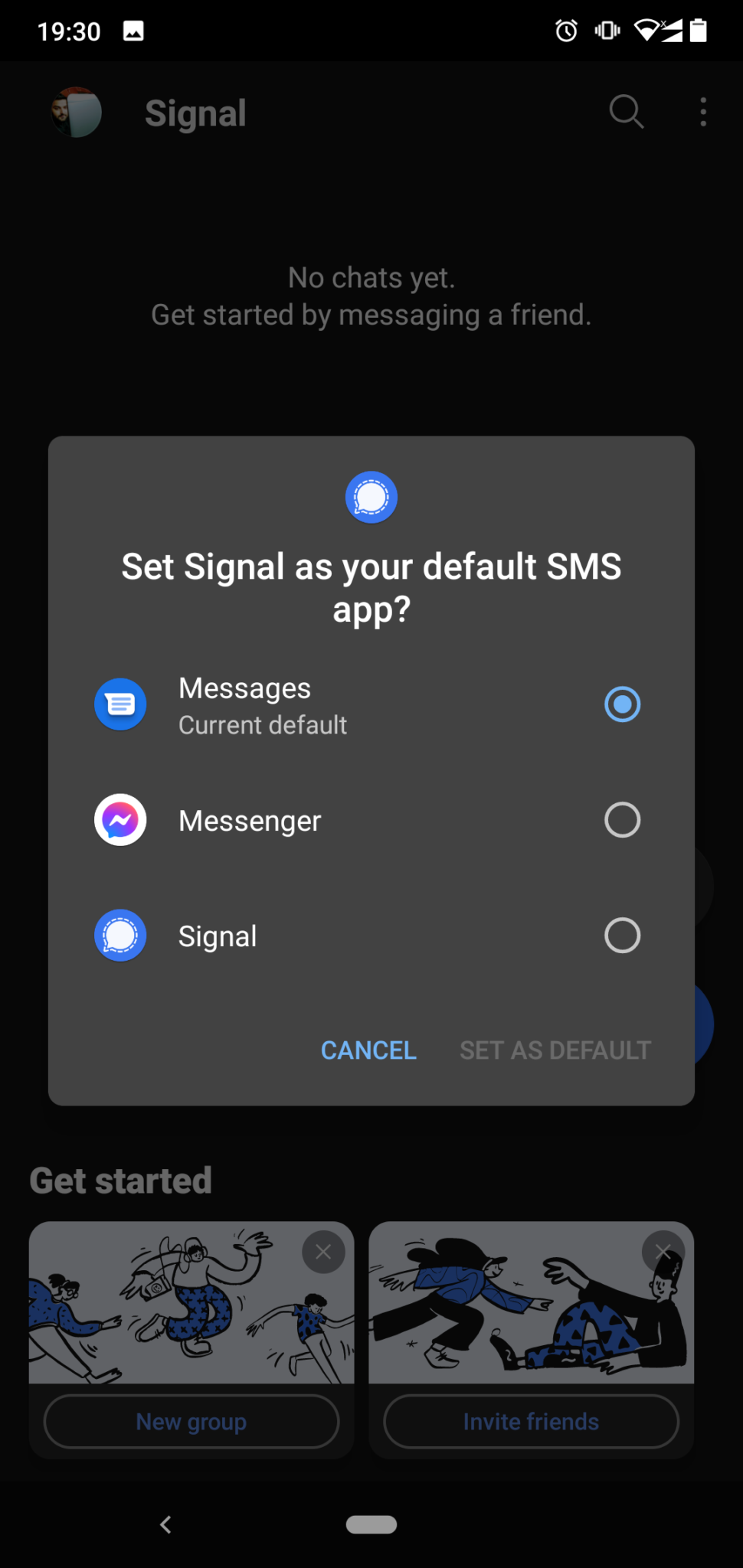This is a detailed screenshot of a phone interface with various elements and indicators visible:

- **Top Bar (Status Indicators):**
  - **Time:** Displayed on the left as "1930."
  - **Notification Icon:** A small white square box to the right of the time.
  - **Alarm Clock Icon:** Positioned to the right, indicating an alarm is set.
  - **Vibrate Mode Icon**: Depicting the phone is on vibrate mode.
  - **WiFi Signal:** Half full, showing a moderate connection.
  - **Unknown Symbol:** A white icon pointing towards the left.
  - **Battery Icon:** A white battery icon, fully charged.

- **Background Text and Elements (Signal App):**
  - **Header:** "Signal" text at the top.
  - **Search Icon:** A magnifying glass icon located on the right of the header.
  - **Main Message:** "No chats yet, get started by messaging a friend," centered on the screen.
  - **Prompt Box:** A gray square in the middle prompting users to "let Signal become your default SMS app."
  - **Message List Options:** Below the prompt, there are options listed as "Messenger" and "Signal."
  - **Buttons:** A blue "Cancel" button in the middle and a "Set as default" button on the right.

- **Bottom Bar (Options):**
  - **Two Photos:** Featured at the bottom, with one on the left and one on the right.
  - **Action Prompts:**
    - Above the photos, there is a prompt saying "Get Started."
    - The left box labelled "New Group."
    - The right box labelled "Invite Friends."

This screenshot signifies a clean, user-friendly interface typical of the Signal messaging app, encouraging new users to get started by setting up default messaging and initiating conversations.